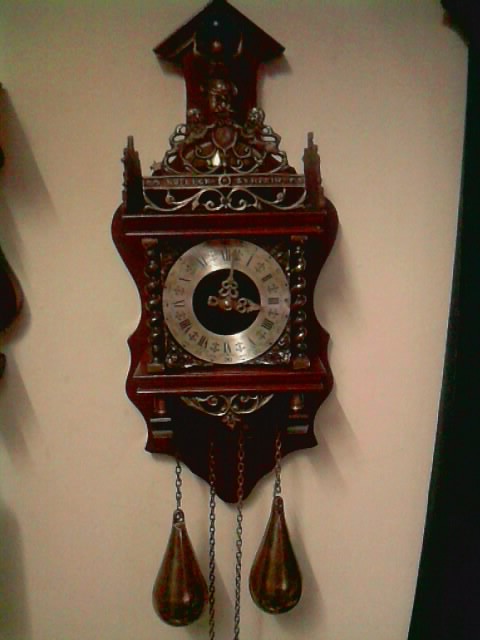This photograph depicts an ornately carved antique wall clock, predominantly made of dark, intricately detailed wood. The clock features a metallic face with Roman numerals and elaborately designed hands, which currently indicate the time as 3:03. At the top of the clock, a small house-like structure adds to its vintage aesthetic, adorned with ironwork curls. The clock is equipped with winding mechanisms, evident from two chains hanging centrally, extending out of the frame. Additionally, there are two heavy, teardrop-shaped weights, resembling boxing practice bags, suspended from two other chains on either side of the central ones, enhancing the clock’s elaborate and functional design. Shadows to the left of the clock obscure an indiscernible object, adding a touch of mystery to the scene.